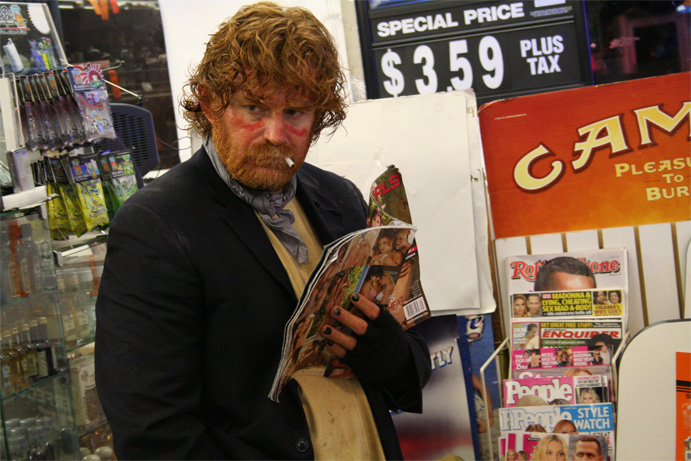In this detailed horizontal rectangular image, a man is standing inside what is likely a gas station or a convenience store, illuminated artificially, indicating the shot was taken at night. This disheveled, rough-looking Caucasian male exudes an aura of disdain with his long, messy orange hair, an unkempt beard, and mustache. His face sports red paint streaks under his eyes, reminiscent of a football player's markings, and he has a cigarette butt protruding from his mouth. His fingernails are painted black, and he is wearing gloves. His attire consists of a dark jacket over a yellow, dirty sweater, which might also include a scarf.

The man holds an open magazine close to his chest but looks away sternly, as if distracted by something off-camera. He appears to be reading a pornographic or celebrity magazine. Surrounding him is a typical gas station display: a magazine rack, advertisements for various products including camel cigarettes, and a clutter of trinkets and quick-buy items. The store's windows reveal the pitch darkness outside, further emphasizing the nighttime setting.